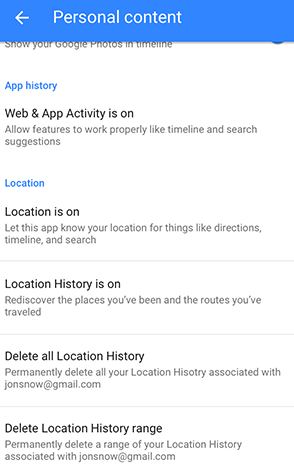This image displays a screenshot of mobile settings related to personal content and activity tracking on Google services:

At the very top of the screen, there is a blue header with a white arrow pointing upwards, labeled "Personal content." Just below this header, an arrow pointing to the left is also displayed in white.

The main body of the screen shows various settings options:
1. Under the blue header, a label reads "Show your Google photos in timeline."
2. Beneath this, another blue label reads "App history."
3. Following that is a black header stating "Web & App Activity is on." In smaller gray text underneath, it explains, "Allow features to work properly like timeline and search suggestions."
4. Next, a blue label reads "Location."
5. Another black header reads "Location is on," with smaller gray text below stating, "Let this app know your location for things like directions, timeline, and search."

A gray divider line follows.

6. The next black text header reads "Location History is on," with smaller gray text underneath specifying, "Rediscover the places you've been and the routes you've traveled."

Another gray divider line follows.

7. The following black header states, "Delete all location history," with smaller gray text below explaining, "Permanently delete all your location history associated with JonSnow@gmail.com."

Another gray divider line follows.

8. Finally, the black header reads "Delete location history range," with gray text underneath stating, "Permanently delete a range of your location history associated with JonSnow@gmail.com."

This detailed outline demonstrates the various settings options related to tracking and displaying personal data within the Google services framework on a mobile device.